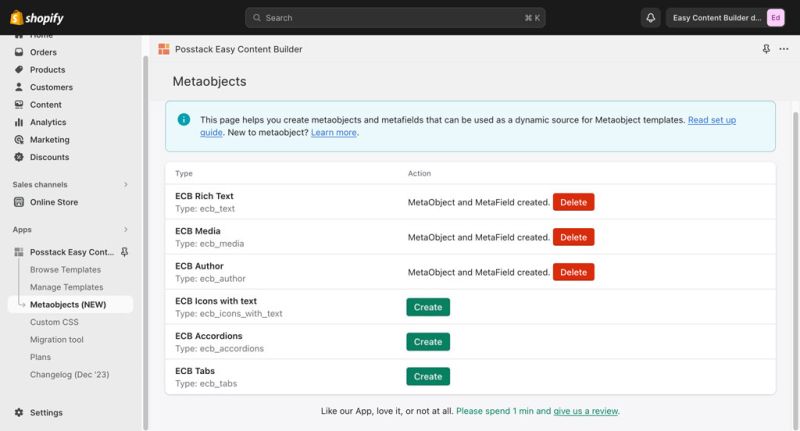This image is a screenshot from the software application, Shopify. The interface shown belongs to the section designated for managing apps and meta objects. Dominating the scene is a primary information box that instructs users on creating meta objects and meta fields, which serve as dynamic sources for meta object templates. The provided text reads, "This page helps you create meta objects and meta fields that can be used as a dynamic source for meta object templates. Read setup guide. New to meta object? Learn more."

The web page features a predominantly light gray and white color scheme, with a top banner that is black. The Shopify logo, accompanied by the word "Shopify," is visible in the top left corner. In the body of the meta objects page, six different headings are presented under the "Type" category. Users have the option to delete the top three headings and create new ones in the bottom three slots.

The overall layout is clean and functional, designed to guide users through the process of configuring their meta objects and fields efficiently.